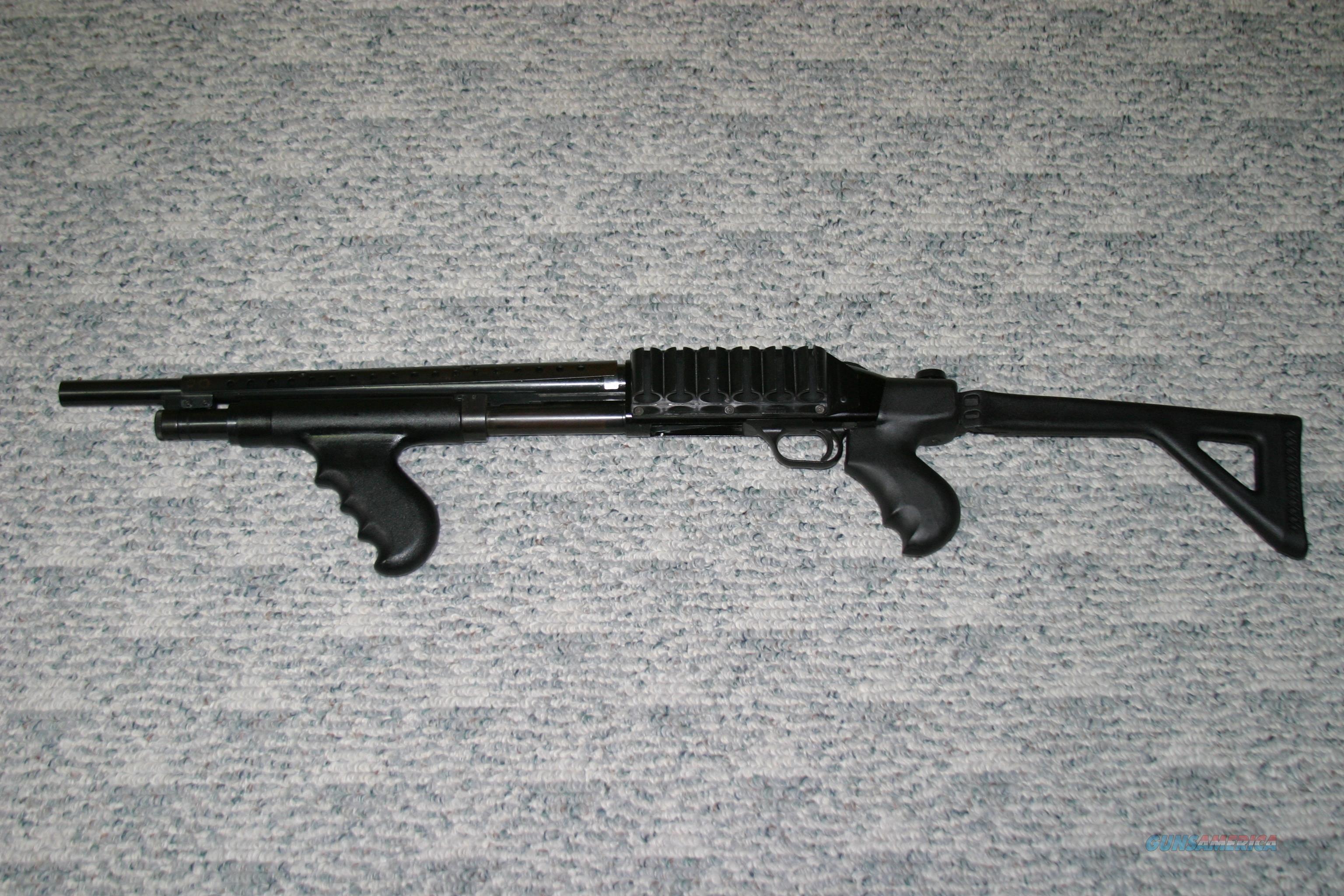The image depicts a black shotgun with shiny accents, centrally placed on a gray and beige carpet with green specks and a faint triangular diamond pattern. The firearm, which appears to be a lengthy pump-action shotgun, has a long body and features two handles. The rear handle includes a triangular stabilizer bar. Above the trigger, there are six slots likely meant for shotgun shells, though none are present. The full barrel is visible, but it's unclear if the gun is loaded or if the safety is engaged. The setting suggests the picture was likely taken indoors, possibly in a residential setting, focused solely on showcasing the shotgun.